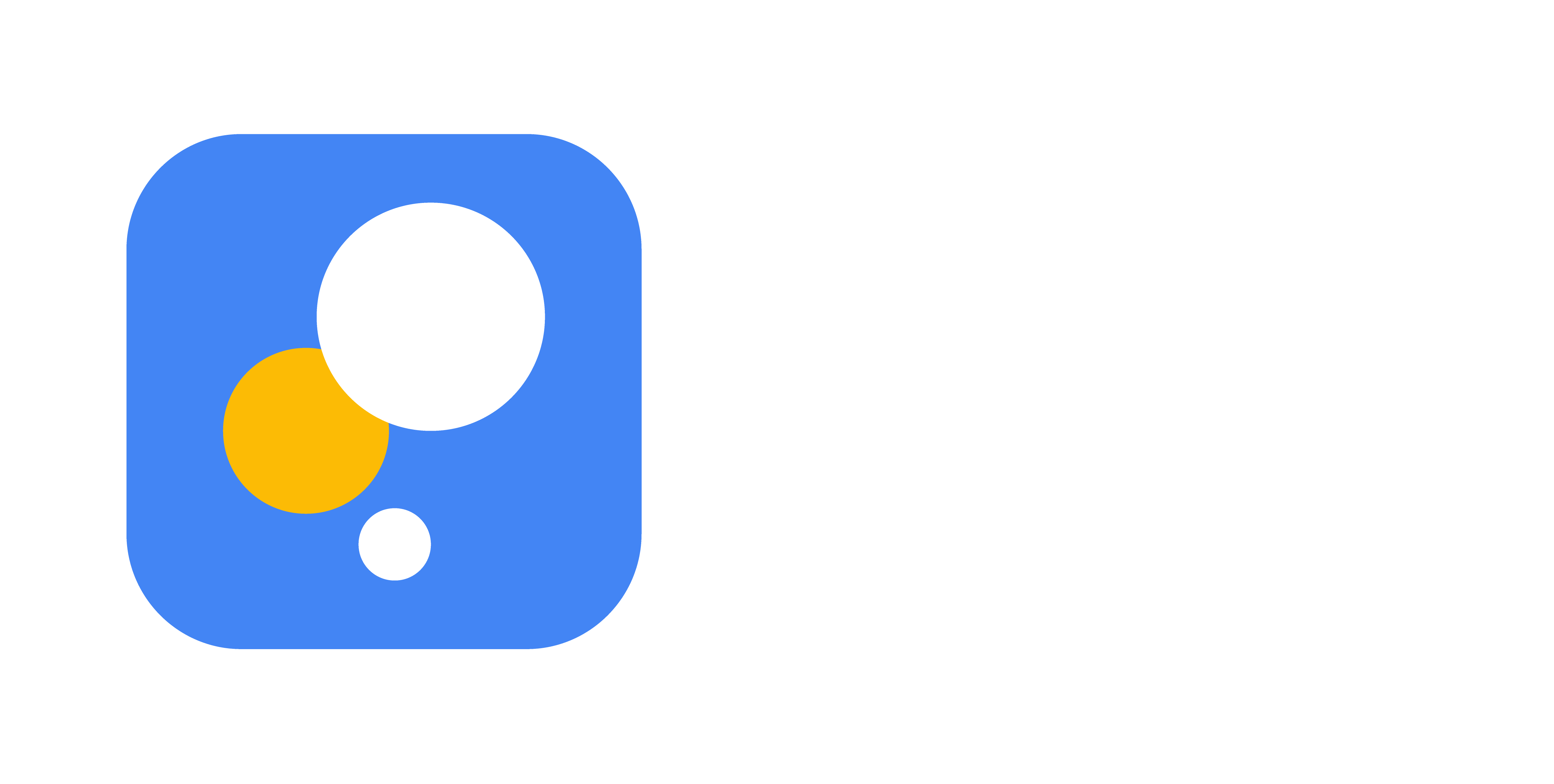The image appears to be a screenshot of an app logo or icon. The icon itself is a rounded square with a blue background. Positioned towards the top right of the square is a large white circle. Below and slightly to the left of the white circle is a smaller yellow-gold circle, and the two circles partially overlap, with the yellow-gold circle being on the bottom. Directly centered below these overlapping circles is a much smaller white circle.